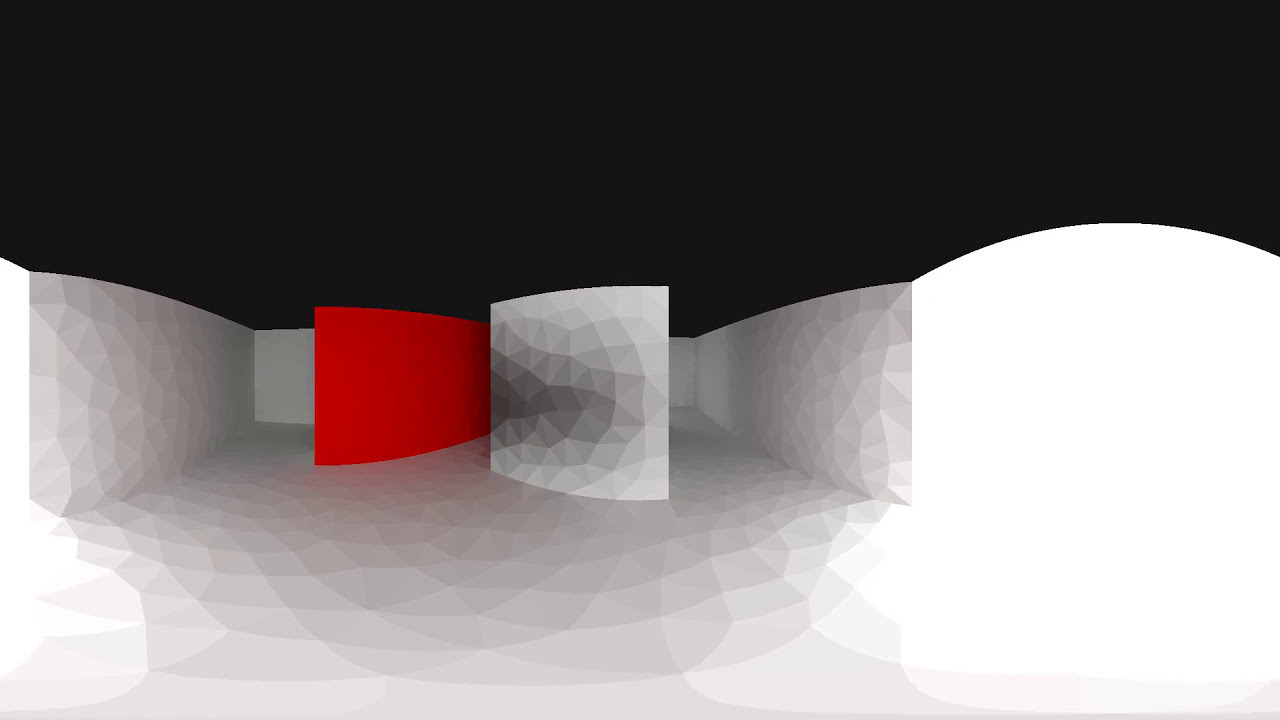This computer-generated artwork, shaped in a horizontal rectangle, features a stark contrast of colors and textures. The upper third of the image showcases a deep black background, resembling a night sky. Below this, the remaining two-thirds of the composition is dominated by a white structure with a textured, ridged surface. This structure, resembling a roofless building, extends across the floor and walls, creating a unified, intricate pattern of geometric shapes, including squares and diamonds.

In the center of the image, there are two prominent freestanding walls. One, located slightly to the left, is a smooth, bright red horizontal rectangle, starkly contrasting with its textured surroundings. To the right of the red wall, there is a vertical white wall section that blends with the building's ridged texture. This white partition features a bold, wide streak that transitions from dark gray to light gray, spanning the middle of the wall. The overall scene is an intriguing blend of sharp contrasts and intricate designs, making for a visually captivating composition.